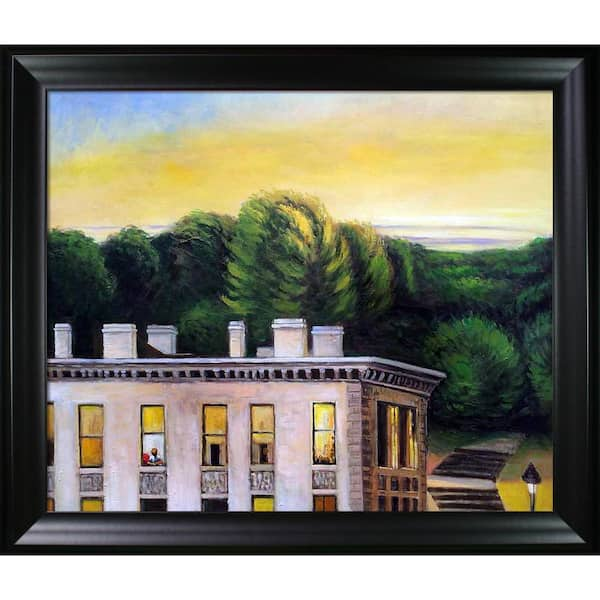The painting, framed in a plain black border, captures an upper story of a modern, pink stone building with numerous chimneys atop its flat roof. The structure, adorned with ornate carvings below its six visible windows, features well-lit, yellow-hued windows in various states; some shades are drawn, while others are opened. In one window, a man in a white shirt is seated on a red chair, providing a glimpse of life inside. Adjacent to the building on the lower right is an old-fashioned streetlamp beside a set of stairs leading to a woodland path, suggesting a connection between the urban setting and nature. The background is dominated by vibrant, wind-swept trees and bushes under a sky filled with the yellow and purple hues of a sunrise, adding to the dynamic atmosphere of the scene.